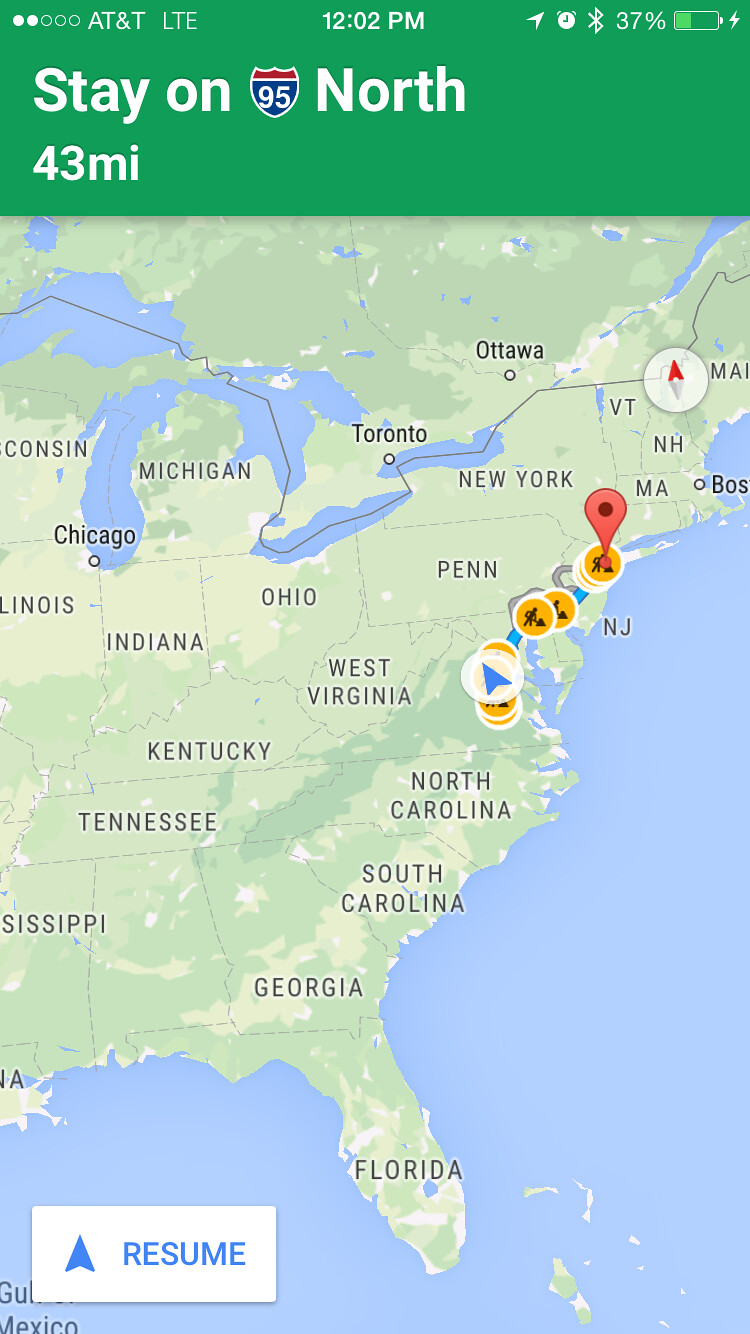This is a color illustration, possibly a screenshot from a mobile phone or tablet, showcasing a detailed map formatted for such devices. At the very top, typical mobile interface symbols are visible, including signal strength, "AT&T LTE", the time "12:02 PM", and a battery life indication of 37%, alongside Bluetooth status. Below this, a green band displays the directive "Stay on 95 North" in white text, with an interstate emblem marked "95" in white and a label "43MI" indicating a distance of 43 miles.

The main portion of the image, occupying roughly 85% of the space, is a map centered on the eastern United States, extending west to include states like Wisconsin, Illinois, and Mississippi, and east to the Atlantic Ocean with parts of Canada visible. Notable states shown include Georgia, South Carolina, Florida, North Carolina, Tennessee, Kentucky, West Virginia, Pennsylvania, Ohio, Michigan, New York, and others. The map delineates a blue route line heading northeast, indicating a drive possibly from Maryland or Washington D.C. to New York City. Along the route, orange circles symbolize construction zones, and a prominent red pin marks the destination, located in New York City. Below the route and to the left, a white rectangle with a blue arrow labeled "Resume" is present. The map is zoomed out, offering a wide perspective of the region, including the Great Lakes and the Gulf of Mexico.